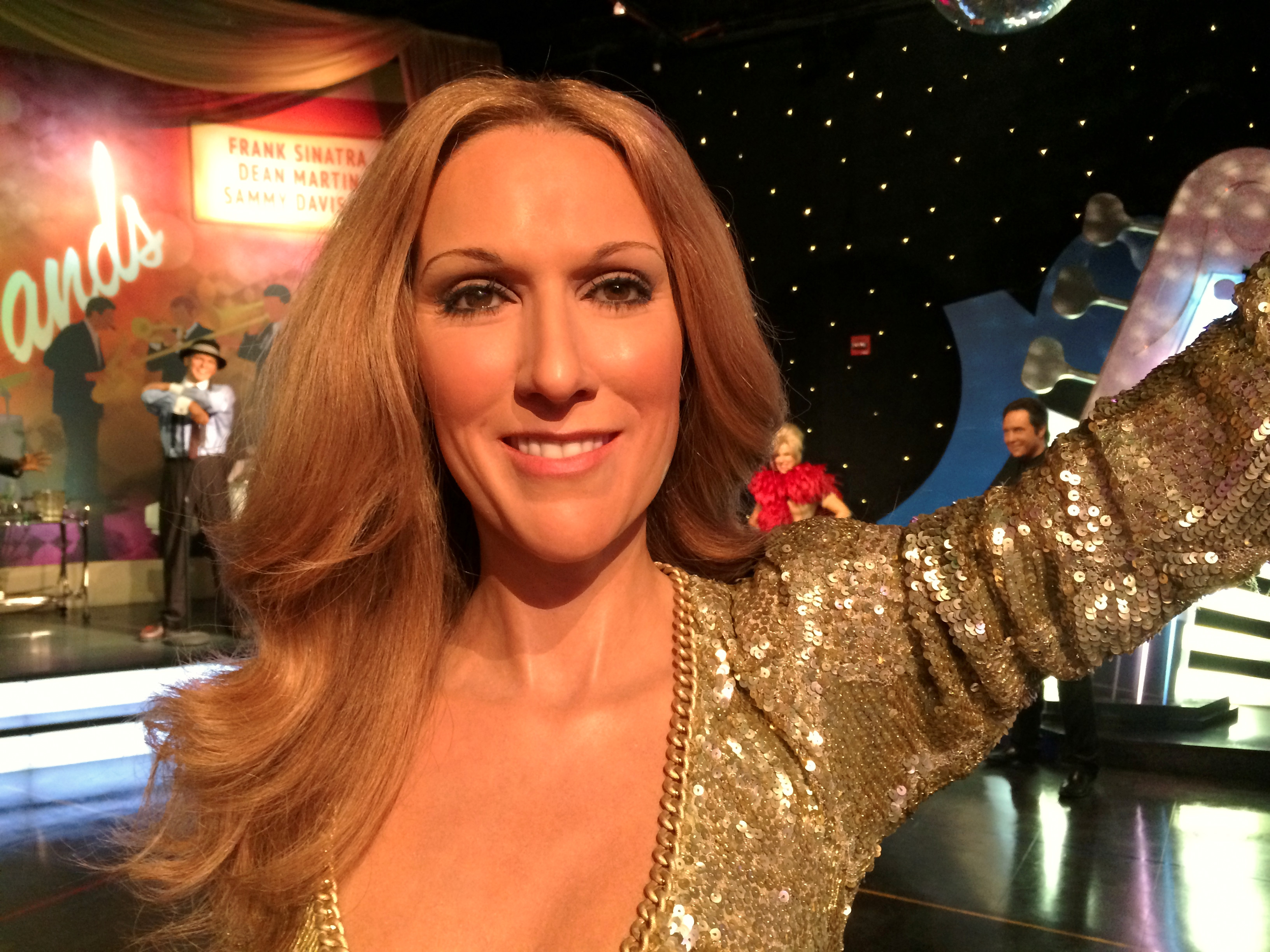This is an image of a wax figure of Céline Dion, prominently displayed at Madame Tussauds in Las Vegas, Nevada. The wax figure is intricately detailed, capturing Céline Dion's likeness with her long, flowing blonde hair cascading to the side. Her lifelike brown eyes and subtle smile reveal the top of her teeth. She is adorned in a glamorous, low-cut, gold sequined dress, with a neckline resembling a gold chain. Céline's left arm is outstretched in the air, adding a dynamic pose to the figure. 

In the background, we observe other wax figures, including those of Frank Sinatra, Dean Martin, and Sammy Davis Jr., positioned on a stage. The backdrop features a starry sky, with small, sparkling dots against a black area, enhancing the scene's theatrical ambiance. The setting is unmistakably part of the Las Vegas exhibit, showcasing these iconic performers in a sophisticated and detailed manner. The photograph provides a close-up view, emphasizing the meticulous craftsmanship of Céline Dion's wax figure.